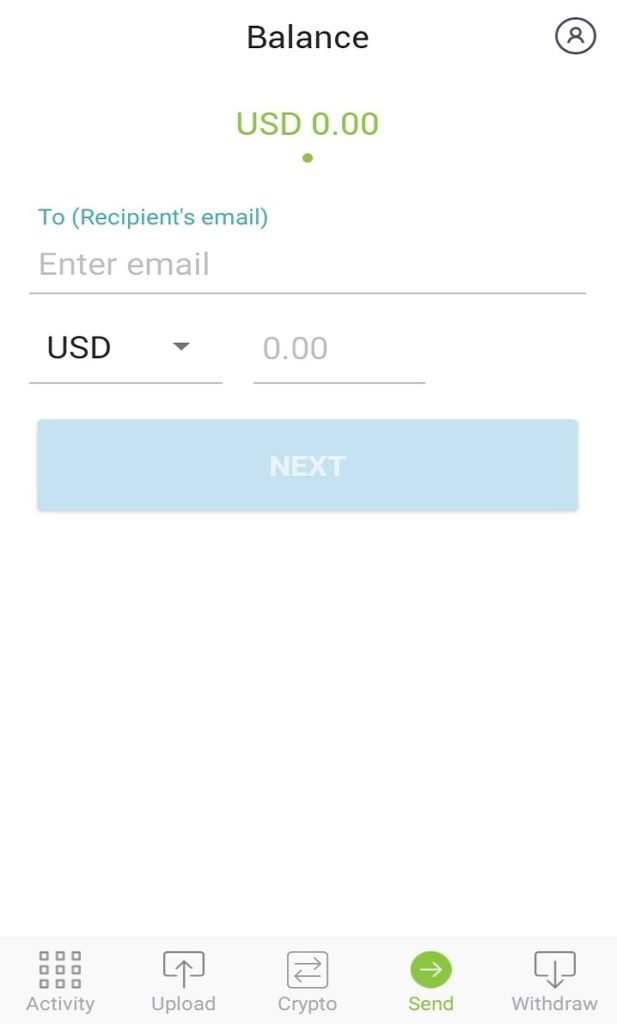This image displays a screenshot from a banking or money transfer app. At the top of the screen, the title "Balance" is prominently displayed in black lettering. In the top right corner, there is a circular icon featuring a simplified stick figure, which likely serves as the account button.

Beneath the title, the balance is displayed in green text, showing "USD 0.00." Below this, the number "2" is followed by "(recipient's email)," leading to a text box where the user can enter the email address of the recipient. There is also a section below for selecting the type of currency, with "USD" currently chosen. A drop-down arrow next to the currency selection allows for changing to a different currency. Below this, there is an input box for entering the amount to be sent, presently showing "0.00." A blue "Next" button is visible but currently grayed out.

Along the bottom of the app, there are multiple tabs arranged in a row. The leftmost tab is labeled "Activity," represented by an icon of nine small squares arranged in a 3x3 grid. The next tab features an upload button, symbolized by a rectangle with an upward-pointing arrow. The "Crypto" tab follows, depicted by a rectangle with two arrows—one pointing left and the other pointing right. The "Send" tab, marked by a round button with a right-facing arrow, is highlighted in green, indicating that it is the currently selected tab. The final tab is the "Withdraw" button, shown by a rectangle with a downward-pointing arrow.